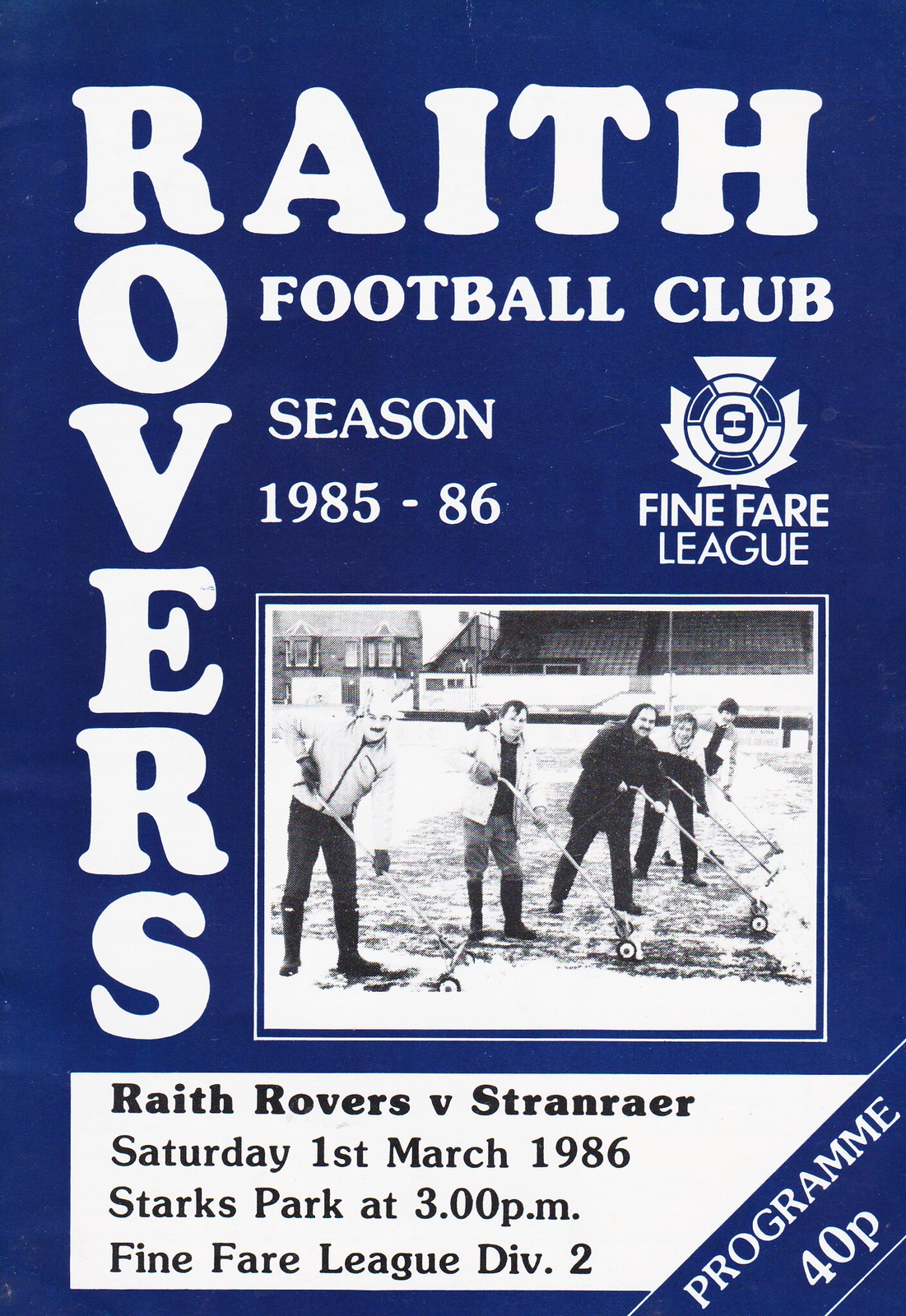This image depicts a detailed poster primarily featuring blue and white colors. At the top, in large white letters, it reads "Raith Rovers," with "Rovers" arranged vertically starting from the 'R' in "Raith." Beneath "Raith" in smaller text, it states "Football Club, Season 1985-86." To the right of the text, there is a logo featuring a soccer ball overlaying a simplistic leaf outline, accompanied by the inscription "Fine Fare League."

Centered on the poster is a black-and-white photograph bordered in white, showcasing five men outdoors on a field. These men appear to be working with small, wheeled devices, presumably snow plows or grass cutters. 

Towards the bottom of the poster, additional text details an upcoming match: "Raith Rovers vs. Stranraer, Saturday 1st March 1986, Stark's Park at 3pm, Fine Fare League Division 2." In the bottom right-hand corner, the cost "Program 40P" is indicated in white capital letters.